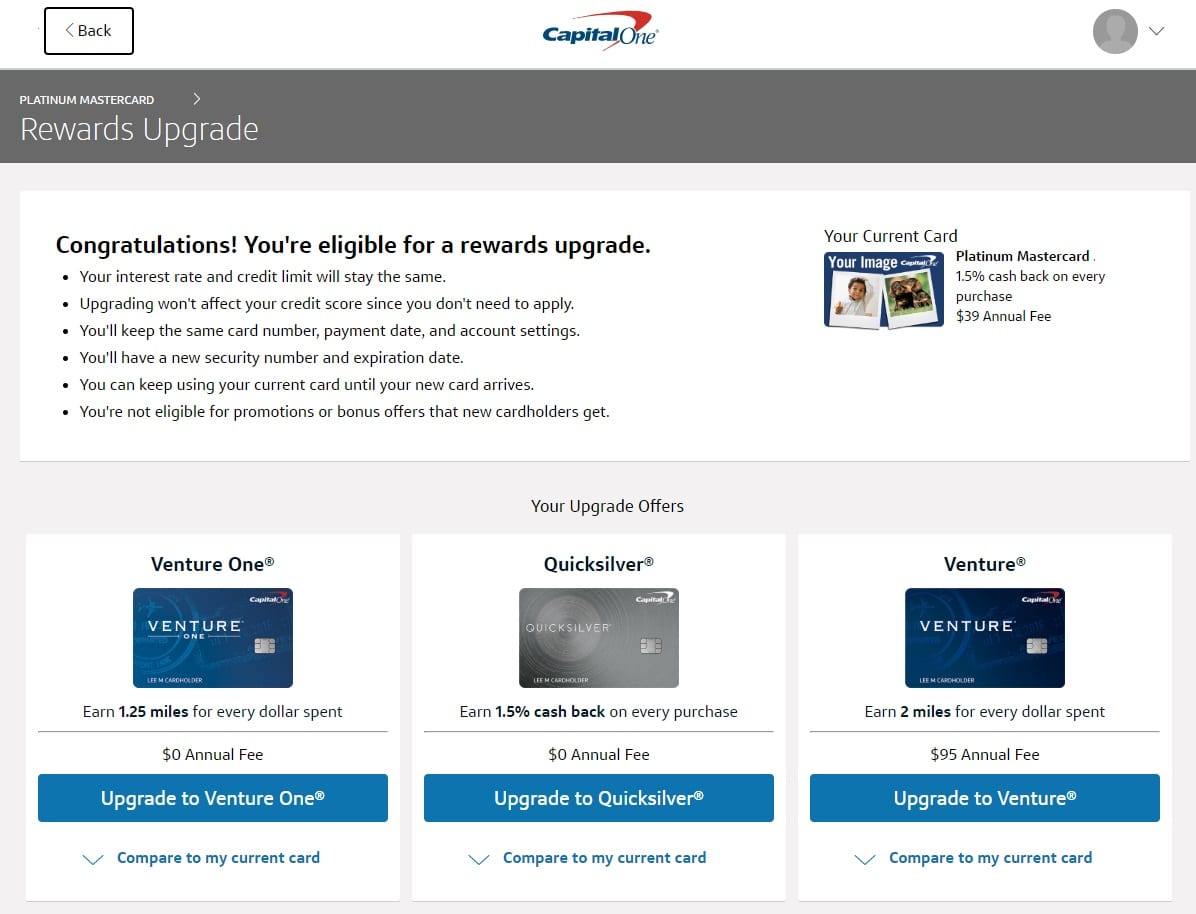**Caption:**

This image showcases a Capital One website page focused on rewards upgrades. The prominent "Capital One" logo, displayed in blue font, features an intersecting orange curved symbol. To the left, there's an outlined black box with a "back" option. On the right, a user icon with a dropdown arrow indicates account information access.

The page centers around rewards upgrades for a Platinum MasterCard, highlighted in a gray rectangle stretching across the webpage. The background is light gray, with various sections delineated by white boxes. At the top, a bolded message in black font congratulates the user: "Congratulations, you’re eligible for a rewards upgrade." Beside this, the current card details are listed.

Below the title, a breakdown of benefits available with the rewards upgrade is itemized in bullet points. Further down, three distinctive white boxes present different credit card options, such as VentureOne, Quicksilver, and Venture, each offering unique upgrade opportunities. The overall design emphasizes clarity and easy navigation for users exploring their reward options.